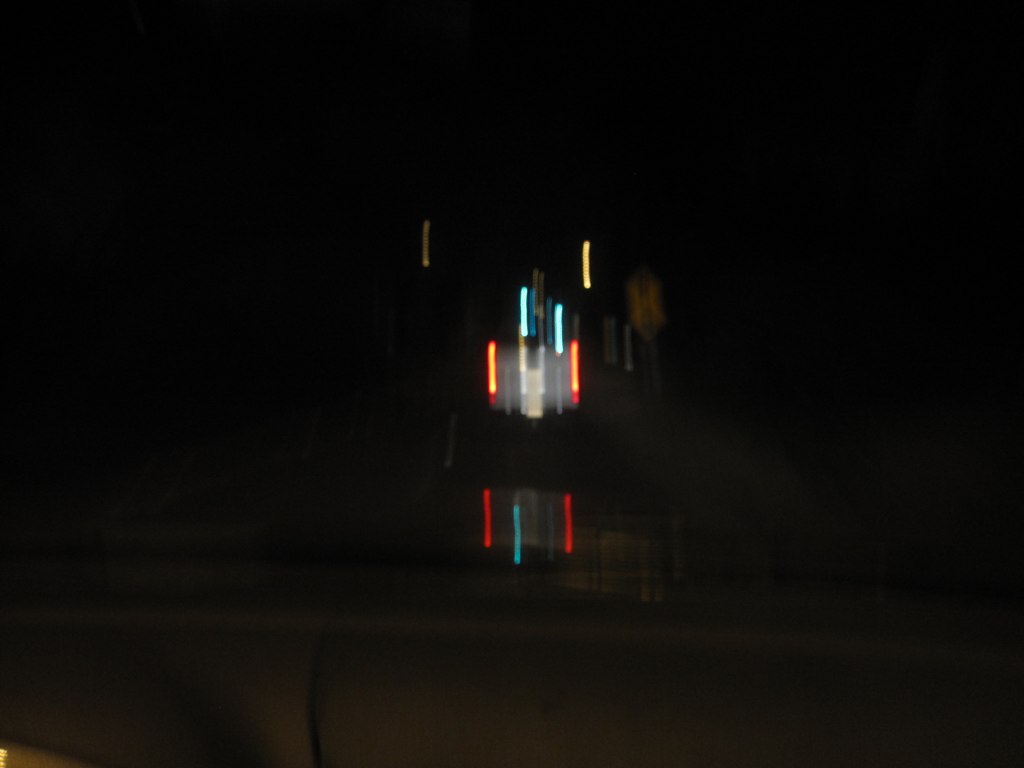The photograph captures a night-time scene through the front windshield of a moving vehicle. The sky is pitch black with no visible stars. The image features a blurry vehicle ahead, its motion accentuated by vertical red and blue streaks of light from the tail lights. These lights reflect off the windshield, reinforcing the motion blur effect that permeates the scene. The background reveals a dark gray interior upholstery of the viewing vehicle. A distinctive yellow and black diamond-shaped traffic sign is visible to the right of the leading vehicle, adding a hint of structure amidst the blended colors and lines.